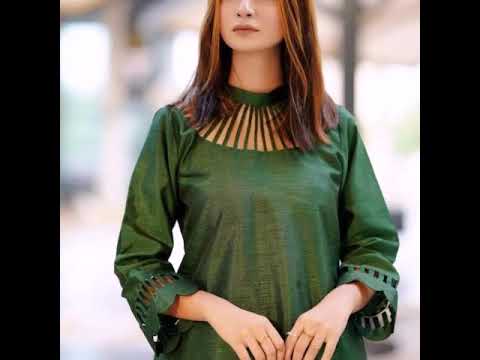This close-up color photograph, likely meant for a clothing advertisement, features a young woman with reddish brown auburn hair cascading past her shoulders. The image captures her from the nose down to about the hip area, with her eyes strategically cut off. She dons a dark green, loose-fitting tunic with a fan-like slitted design around the neckline and bell sleeves that mirror this motif with peek-a-boo slits at the elbows. Her hands, adorned with a couple of rings on her left hand, are positioned with her index fingers touching in front of her abdomen. She maintains a neutral, pleasant expression against an out-of-focus background that suggests an urban outdoor setting. The photograph is bordered with a black stripe on each side, adding a framing effect to the overall composition.